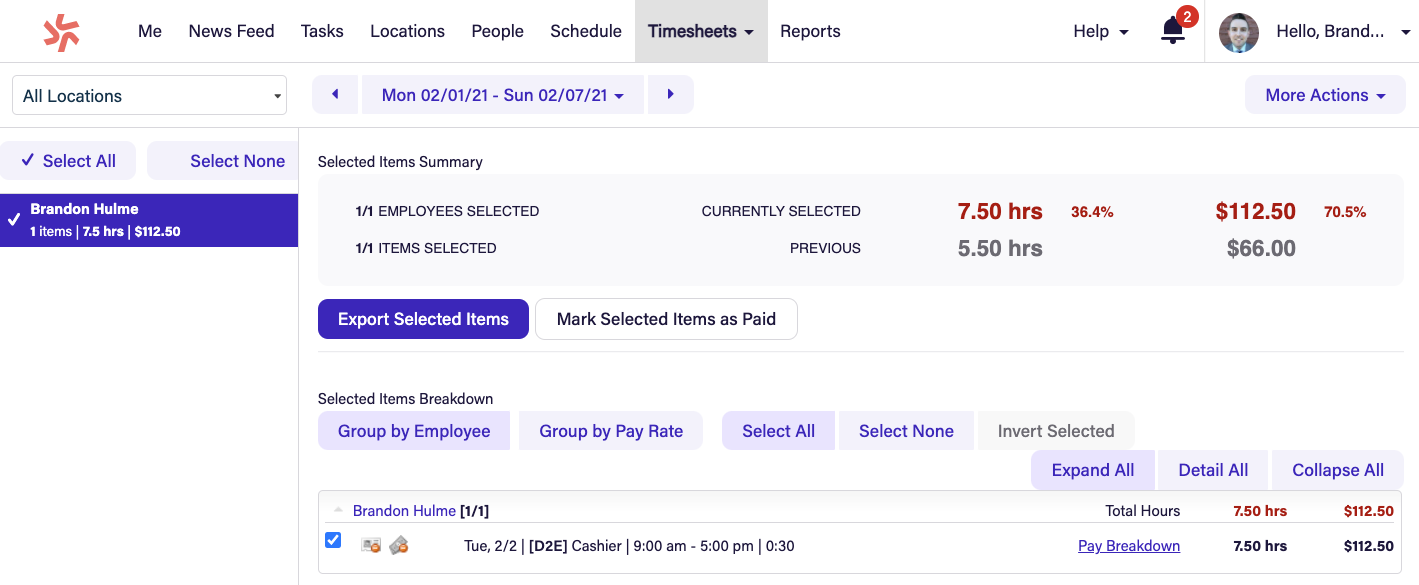The webpage displays a predominantly white background in the top left corner, accentuated by an orange icon featuring three "V" shapes oriented in different directions. Adjacent to the icon is a vertical menu in black text listing various options: "Me," "Newsfeed," "Tasks," "Locations," "People," "Schedules," "Timesheets," and "Reports." The "Timesheets" option is selected, indicated by a light gray rectangle surrounding the bolded text.

Below the menu, there's a section for location selection, starting with "All locations" followed by a dropdown menu. Within this dropdown, the options "Select All" and "Select None" are displayed on light purple, rounded rectangular backgrounds. Continuing down, the name "Brandon Hume" (spelled "H-U-L-M-E") is listed with "one items" beneath it. Following this, two dividers section off the text "7.5 hours" and the amount "$112.50," all set against a dark purple background with white text.

To the right, a "Selected Item Summary" is presented in black text. Below this heading is a long rectangular light gray area containing black text that reads "1/1 employee selected, currently selected." In bold red text, it states "7.50 hours," accompanied by smaller bold red text showing "36.4%." Further bold red text displays "$112.50," with smaller text indicating "70.5%."

At the very top right, there's a help option with a dropdown menu, alongside a black bell icon with a white number "2" in a red-filled circle, signaling two notifications.